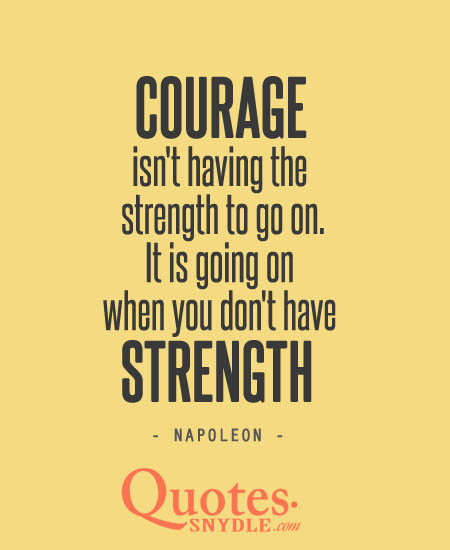This color image, resembling a meme or an inspirational quote often seen on social media platforms like Facebook, features a canary yellow background. Prominently displayed in the center is the motivational message. The text begins with the word "COURAGE" in all capital and bold black letters. The message continues with "isn't having the strength to go on. It is going on when you don't have strength." The word "STRENGTH" is also emphasized in bold black letters. This quote is attributed to Napoleon. At the bottom of the image is an orange logo for "QuotesSnydel.com," highlighting the source.